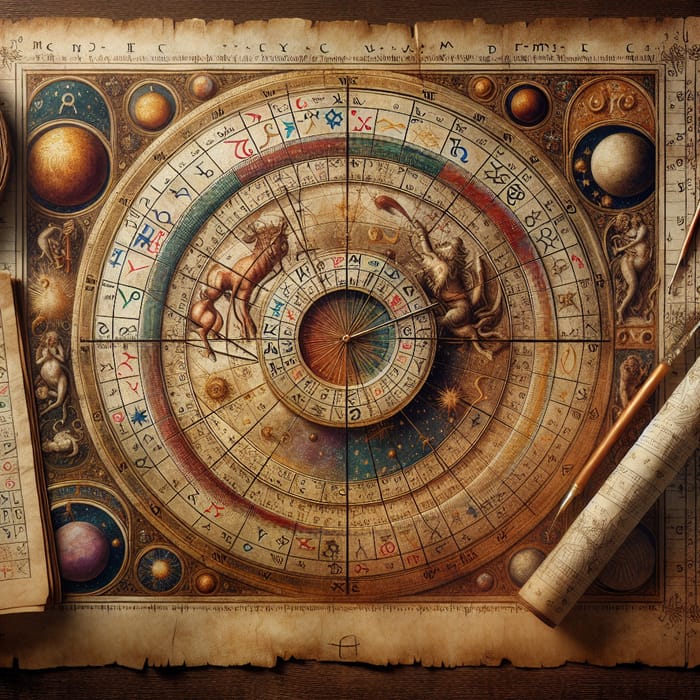This image presents an intricate design on an aged piece of parchment, exuding an antiquated and mystical feel. Central to the illustration is a large, multi-layered circular mechanism reminiscent of a sundial or ancient calendar. It features several concentric circles segmented with black lines, adorned with various intricate symbols and hieroglyphic-like markings. The central circle houses a needle or hand, which points diagonally, suggesting it might measure something, but not necessarily time. The area around the needle contains alternating bands of colors—red, green, and tan—each section filled with distinctive symbols. 

Encircling these sections are images of animals, notably a monkey and a bull, and stylized human figures, suggesting a cosmic or astrological purpose. The parchment is bordered by depictions of celestial bodies—planets in varying colors such as orange, brown, purple, and gold—on a stark black background, enhancing the celestial theme. Among these, the top left corner is dominated by a series of planets, including distinct orange and brown ones, while the bottom left corner mirrors this with additional celestial bodies.

Accompanying the parchment are various scholarly tools, including an old book that edges into the left side of the image, a rolled-up scroll in the bottom right, and an orange writing instrument nearby, indicating a historical or academic setting. The parchment, with its elaborate design and symbolic richness, appears to be a fusion of an ancient astronomical instrument and a cultural artifact, perhaps akin to a Mayan calendar, embedded in a scene replete with scholarly exploration.